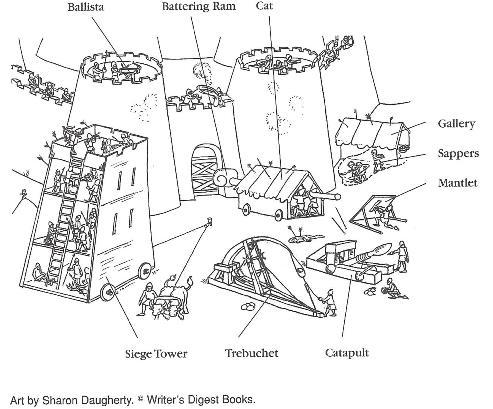This detailed black-and-white hand-drawing by Sharon Daughtry, featured in Writers Digest Books, depicts a dynamic siege against a medieval castle. The scene illustrates various siege weaponry and tactics meticulously labelled for clarity. On the castle walls, defenders operate ballistas, large crossbows shooting foot-long arrows, while archers stand ready at the turrets. The attackers employ numerous contraptions: catapults and trebuchets launch rocks at the fortress, a siege tower—a mobile structure on wheels—allows assailants to scale the walls, and a battering ram targets the gates. For protection, mantlets, large shields with arrow slits, are used, alongside a gallery, which acts as a covered gathering area. Sappers attempt to undermine the castle by digging tunnels. This intricate sketch, blending both artistic and technical elements, vividly captures the intense and multifaceted efforts of a medieval siege.